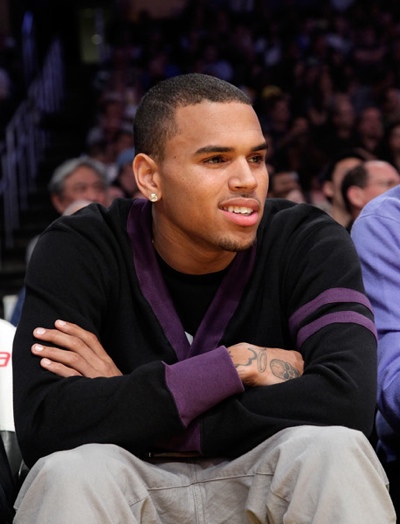This detailed image captures an African-American man, potentially a celebrity such as Usher or Chris Brown, with a caramel complexion, seated amidst a blurry background of an audience, possibly at a sporting event or concert. The man, who appears to be the main focal point of the photo, is dressed in a striking black sweater featuring distinctive purple accents—purple lining around the collar, cuffs, and two purple stripes on his left arm. A black shirt peeks out from underneath the sweater. He complements his outfit with light khaki or beige-colored pants. Notably, a diamond earring adorns his right ear, and there is a visible tattoo on his right hand. With his arms casually crossed and a confident, slightly cocky smirk on his face, he gazes off into the distance to the right of the image. The image captures his poised and relaxed demeanor, with a blue sleeve from another person partially in frame to his left, adding context to the crowded, lively atmosphere.